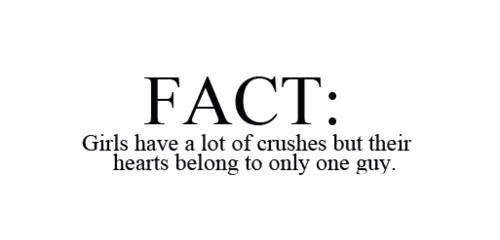The image features a stark white background with centered black text. At the top, in large bold all-capital letters, the word "FACT:" is displayed prominently. Below this, in smaller block lettering, are the words: "Girls have a lot of crushes, but their hearts belong to only one guy." The message is centered and the text style remains consistent throughout. The simplicity of the design, with its dominant white space and black text, draws direct attention to the statement, emphasizing its content without any distractions.